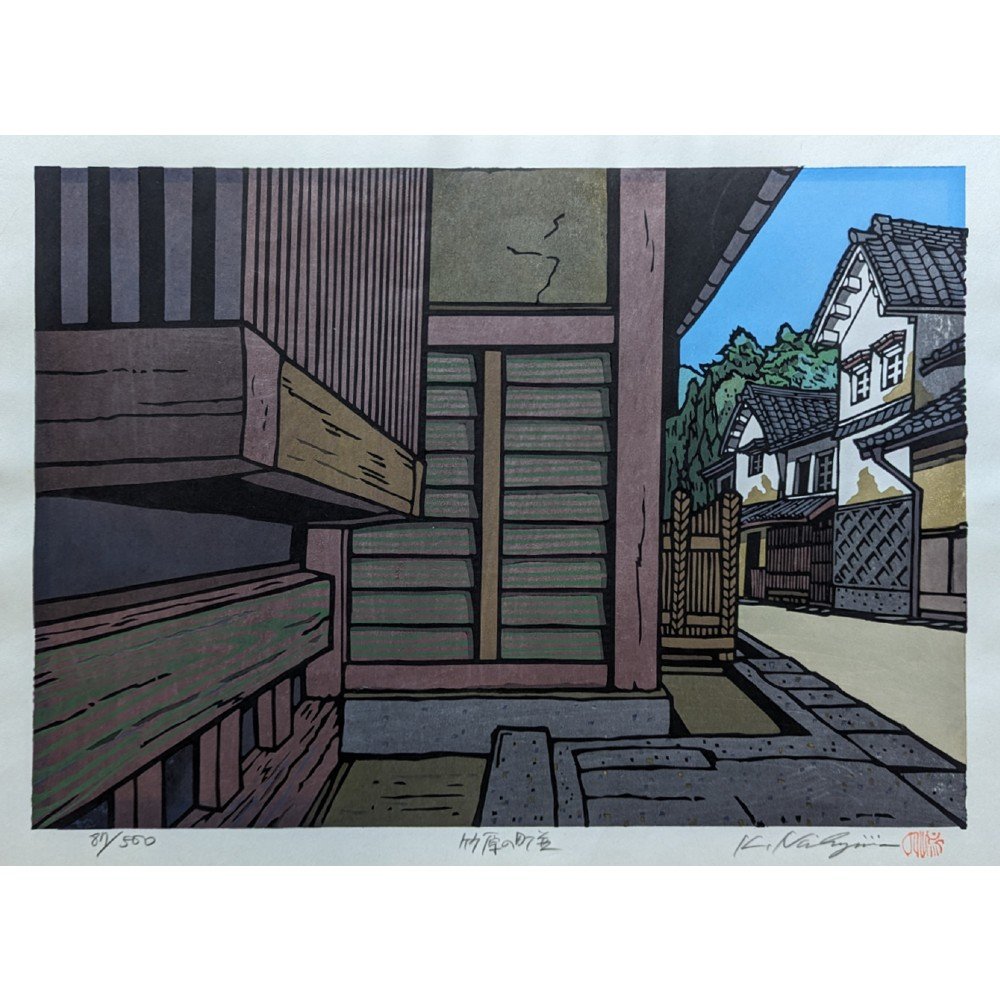This image is a cartoonish illustration, numbered 87 out of 500, depicting a cozy scene in a village. The artwork shows a residential street with a couple of white houses featuring gray roofs and wooden shutters. There are various wooden structures, including a balcony with wooden blinds and a wooden fence, along with some brown staining on the sides of the houses. Across the street, we see a full house, but we only get a partial view of the structure from which the observer might be looking, suggesting the artist's intent to evoke a feeling rather than capture the entire village. The scene is set under a clear blue sky, adding a serene atmosphere. Notable details include a thin gray border around the print, accompanied by the artist's signature—starting with the letter "K" and possibly followed by "N"—as well as some writing possibly in an Asian language along the lower center border, highlighting the artwork's fine-art quality suitable for framing.